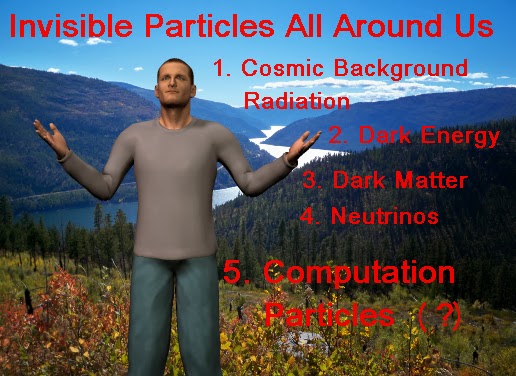This is a detailed illustrative graphic depicting a computer-rendered man in a long-sleeved gray shirt and blue jeans, standing in a grassy field adorned with flowers. The man's arms are raised in a questioning gesture. The backdrop showcases a picturesque, realistic nature scene with a river flowing between lush, green, forested hills and distant mountains under a serene blue sky dotted with white clouds. Superimposed in red text, the image is headlined "Invisible Particles All Around Us," and lists:

1. Cosmic Background Radiation
2. Dark Energy
3. Dark Matter
4. Neutrinos
5. Computation Particles (?)

The words, rendered in a vivid red font, stand out against the tranquil, natural background, creating a powerful juxtaposition between the unseen scientific concepts and the visible beauty of the natural world.